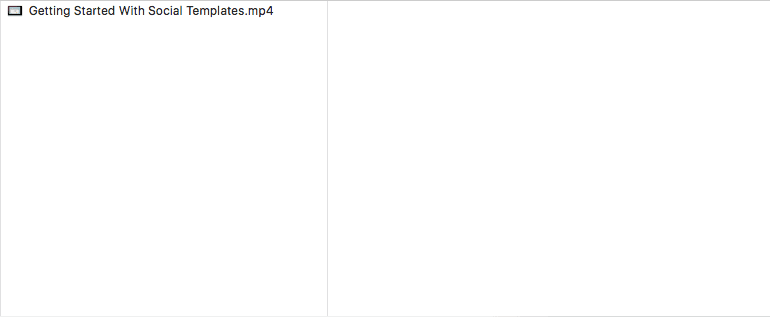The image features a predominantly white background with subtle gray borderlines. Positioned on the left side of the image, there is text in black, specifically at the upper section, which reads "Getting Started with SocialTemplates.mp4." Adjacent to the left edge of the image is a small icon, reinforcing the instructional nature of the content. The text and icon suggest that the image pertains to a video tutorial or guide, likely aimed at assisting users in navigating or utilizing the SocialTemplates website effectively.